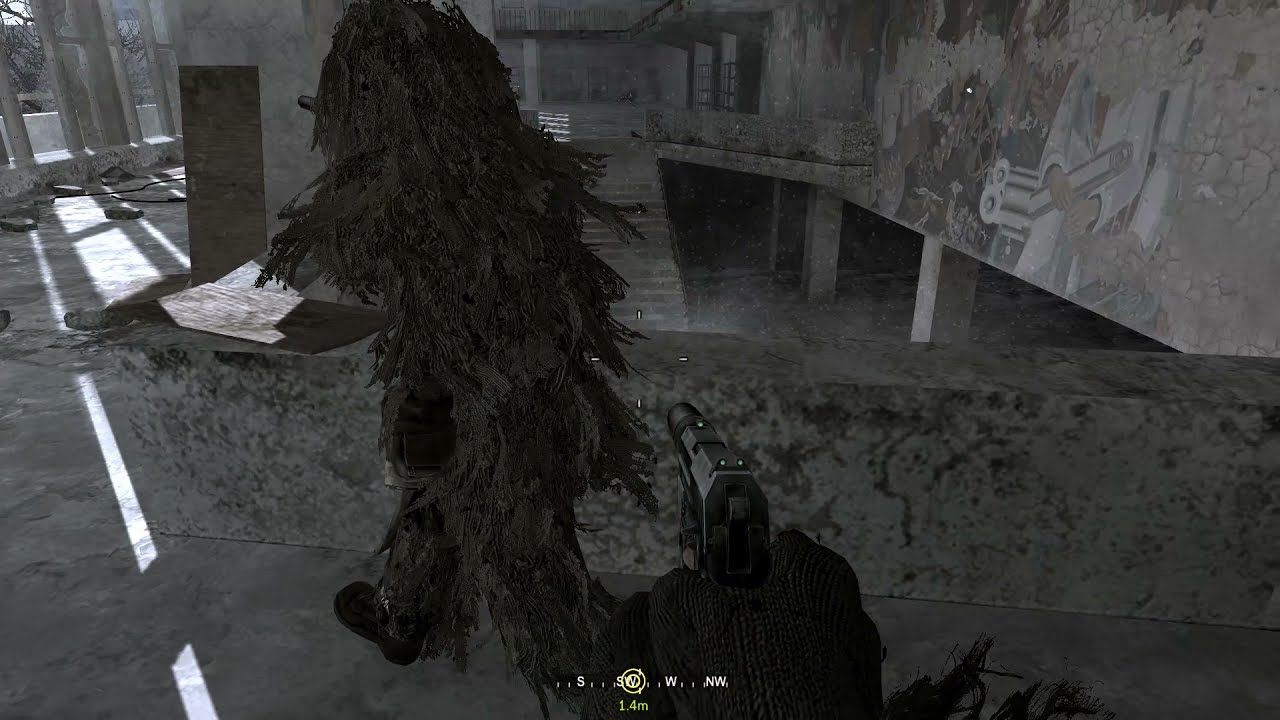In a dimly lit, concrete environment resembling an abandoned building, the picture captures a dramatic moment from the perspective of someone holding a black gun, their hands clad in black fingerless gloves. In the middle ground, a person is walking away from the shooter, dressed head-to-toe in camouflage gear that mimics tree branches, giving an impression of a moving tree or a Sasquatch-like figure. The person wears dark footwear—either black sandals or boots—and appears to be mid-stride on a concrete floor. To the right, there are gray walls adorned with graffiti or murals, and an open dark doorway partly painted in white lets sunlight beam through, highlighting various gray and white areas. A set of gray stairs is visible, leading down into a basement area supported by square concrete posts. Light streams through openings between the columns, illuminating the space. The bottom part of the image includes numeric and directional text, "S, W, NW, and 1,4M," possibly indicating coordinates or measurements important to the context. This scene, likely a snapshot from a video game, combines elements of potential danger with an eerie, post-apocalyptic ambiance.